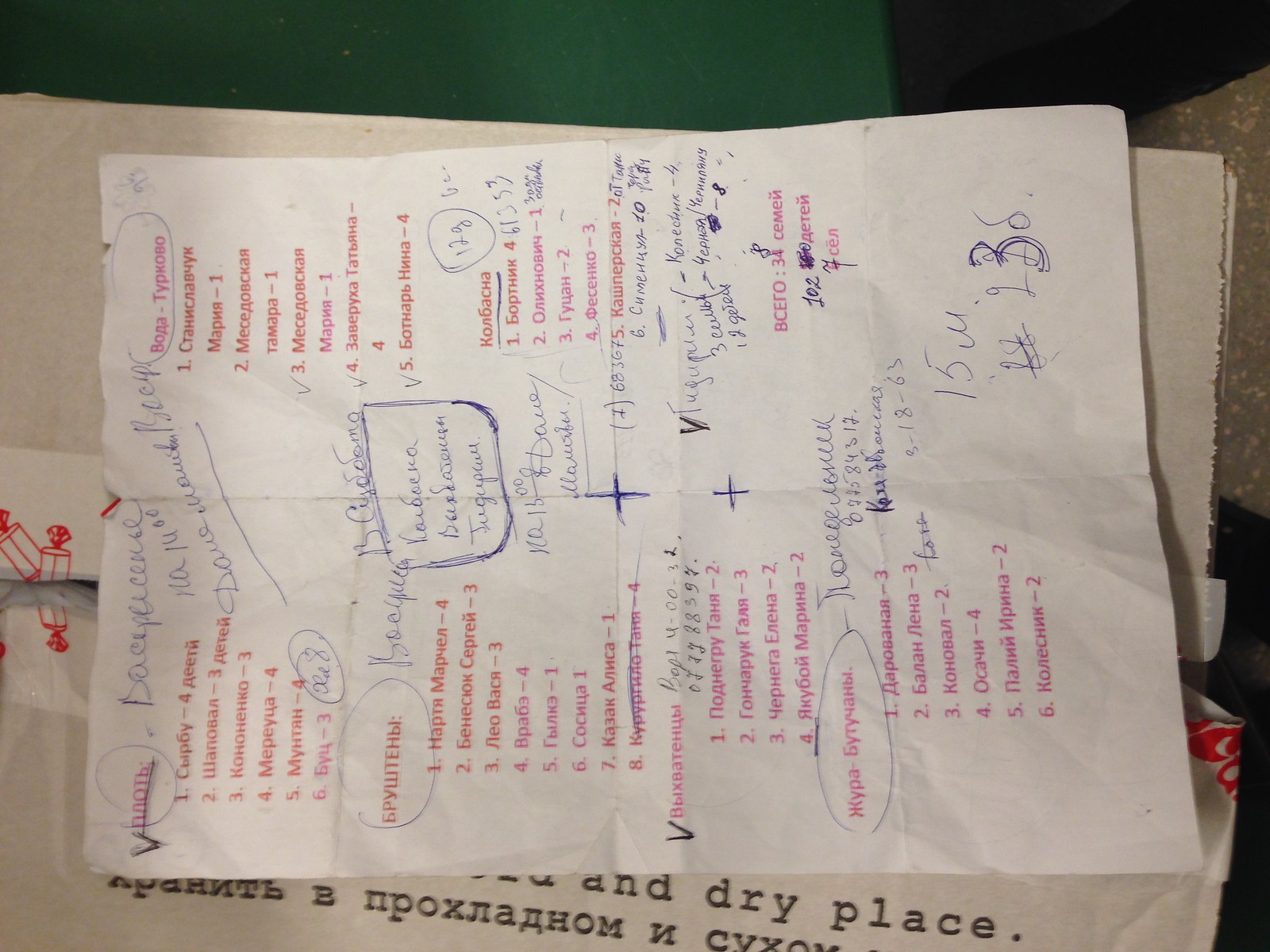This is a full-color photograph of a crumpled piece of paper, turned sideways, making it difficult to read. The paper features red and pink typed text alongside numerous blue handwritten scribbles and notes, indicating heavy annotation. The text appears to be in an unfamiliar language, possibly from the Middle Eastern or Russian regions, which complicates understanding the content. The paper lies on top of a box with legible English text about storing it in a 'dry place,' and some additional text in what looks like Russian. The indoor setting is suggested by the general background, which does not contribute much additional context. The condition of the paper, with its many folds and crumples, further implies it has been handled and reviewed extensively, possibly akin to a school report marked up by a teacher for revisions.